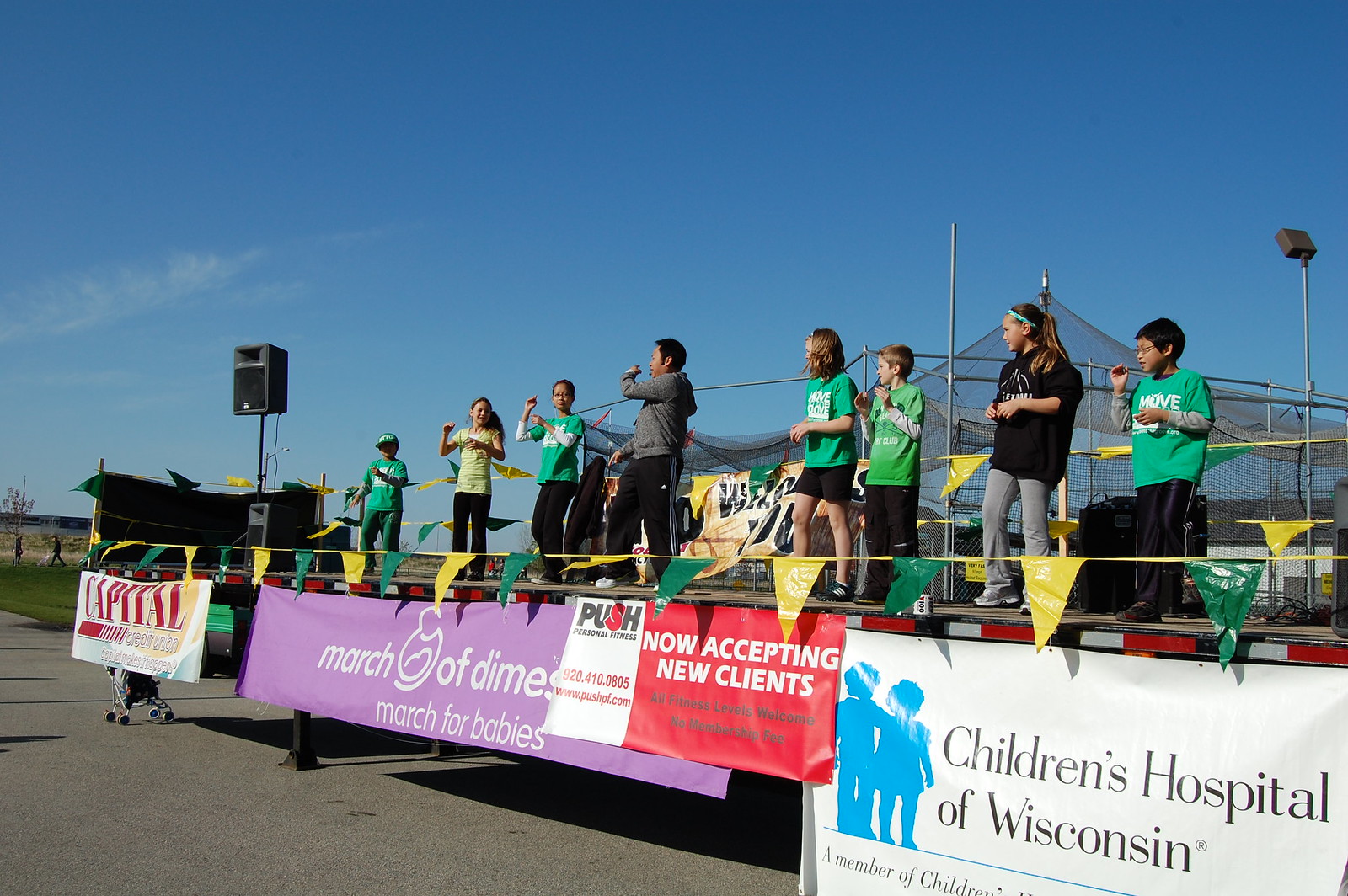The photograph depicts a small event taking place on a makeshift stage, likely an outdoor community gathering or charity event. The stage appears to be slightly elevated and is covered with advertisements and banners. Dominantly, a large purple sign in the center reads "March of Dimes, March for Babies" in white text, indicating the event's affiliation. Surrounding this central banner, additional signs, including a white and red one announcing "Now Accepting New Clients" and a white sign with blue silhouettes declaring "Children's Hospital of Wisconsin," are also visible.

On the stage, a diverse group of about eight individuals, including numerous children clad mostly in green attire, engage with the audience. A man with dark skin and hair, dressed in a gray sweater and jogging pants, stands at the center holding a microphone, possibly leading or announcing to the crowd. Some people appear to be dancing, adding a lively atmosphere to the scene.

The front of the stage is adorned with a row of alternating yellow and green ribbons. The backdrop includes a chain-linked netting and a bright blue sky with minimal cloud cover, suggesting a pleasant day. Speakers or spotlights are set up around the stage to aid in the event's presentation. The overall setting is one of community involvement, celebration, and charitable activity.